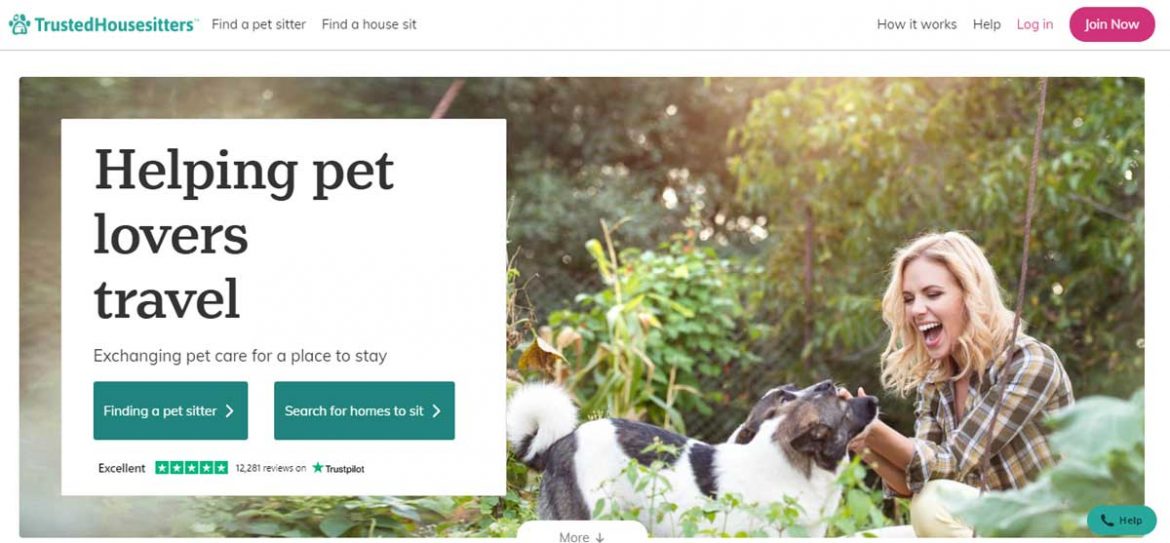The image depicts the homepage of the website "Trusted House Sitters," designed to connect pet lovers with opportunities to care for pets in exchange for accommodation. The central visual features a blonde woman, clad in casual attire, seated outdoors amidst lush, green foliage. She is engaged in a warm, interactive moment with a dog, both gazing at each other affectionately. 

Above the image, there's a white informational box summarizing the site's purpose: helping pet sitters travel by exchanging pet care for a place to stay. The site's navigation options are displayed prominently, including buttons titled "Find a Pet Sitter," "Find a House Sit," and "How It Works," all in green with white text.  

An overlay in the top right corner showcases the site's excellent ratings, flaunting green stars and a notable 1,281 reviews on Trustpilot. There's also a green button with a black phone icon labeled "Help" for customer assistance. 

The call-to-action "Join Now" button stands out in red, urging new users to register. The overall layout features a combination of black and green fonts, complementing the site's cohesive and inviting aesthetic.

Trusted House Sitters is clearly displayed as the website's name, emphasizing its trusted community of pet sitters and pet owners globally.